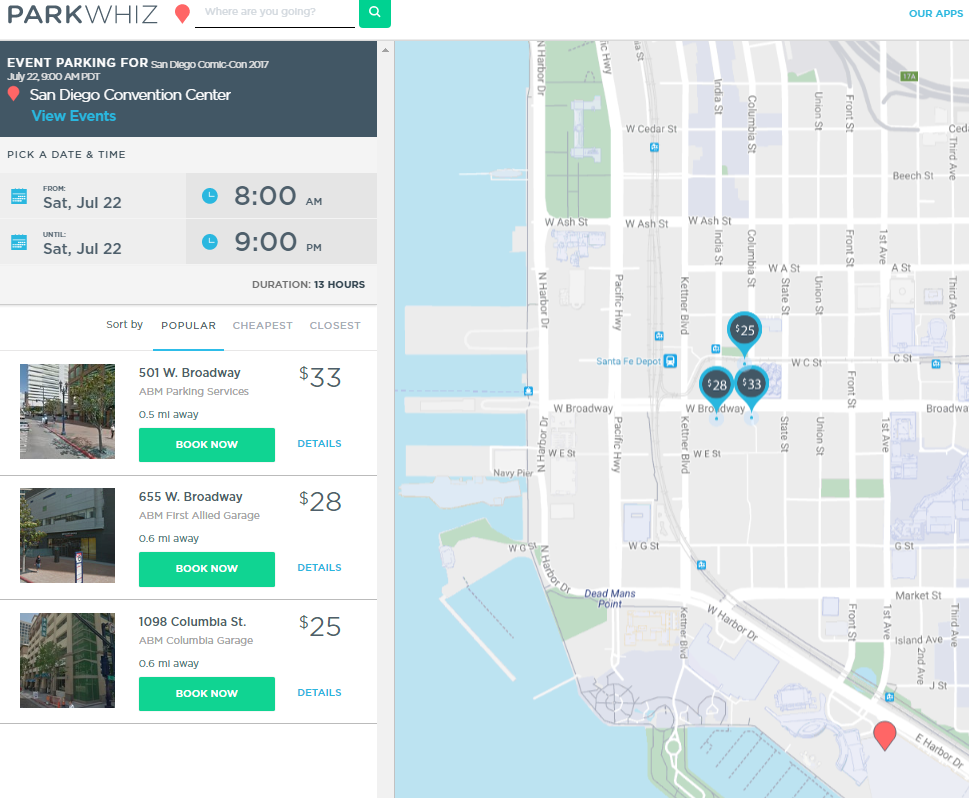**Descriptive Caption:**

The image features a screenshot of a digital map from ParkWiz, prominently shown in the upper corner. The interface begins with a search field displaying the faint prompt "Where are you going?" Positioned below, a dark bluish-gray banner announces in white text: "Event Parking for San Diego Comic-Con 2017," followed by the date and time, "July 22nd, 9 a.m. PDT."

Descending from the banner, the map highlights a single red-marked location—the San Diego Convention Center. Below this, a blue clickable link labeled “View events” is visible. Further down, a field titled "Pick a date and time" offers two options: firstly, from Saturday, July 22nd, 8 a.m. to Saturday, July 22nd, 9 a.m., and secondly, a 13-hour duration window.

Beneath these fields, the image displays three sections with photographs of different parking locations. The first parking option is for "501 West Broadway - ABM Parking Services," priced at $33 and located 0.5 miles away. A green button for booking a parking spot is placed below this first section. The second option is "655 West Broadway," offered at a slightly lower cost of $28 and situated 0.6 miles away. The third option presents "1098 Columbia Street - ABM Columbia Garage," priced at $25 and similarly 0.6 miles away.

Accompanying the textual information, the adjacent street map includes markers. A waterway runs along the map's edge, with small blue and dark blue balloons indicating the three parking locations.